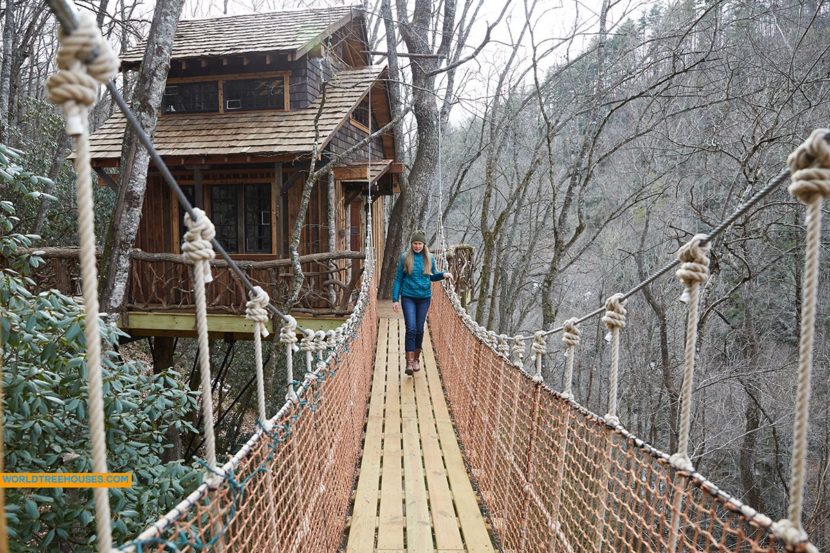In this wide, vertical rectangular image, a young woman with long blonde hair is captured walking across a rope bridge with a wooden plank walkway. She is dressed warmly in a blue jacket, blue jeans, brown boots, and a gray beanie hat. The setting is outdoors, in the midst of a deciduous forest during winter, evident by the bare gray tree trunks and the cold, whitish-gray sky in the background. On the left side of the image, there's some green shrubbery in the foreground. The bridge stretches from the camera's viewpoint to a rustic, brown wooden tree house nestled among the tree trunks. The tree house features two stories and a shingled roof, supported by stilts. The woman is making her way toward the camera, holding onto one side of the rope railing. The lower left corner of the image displays a website link: worldtreehouse.com.